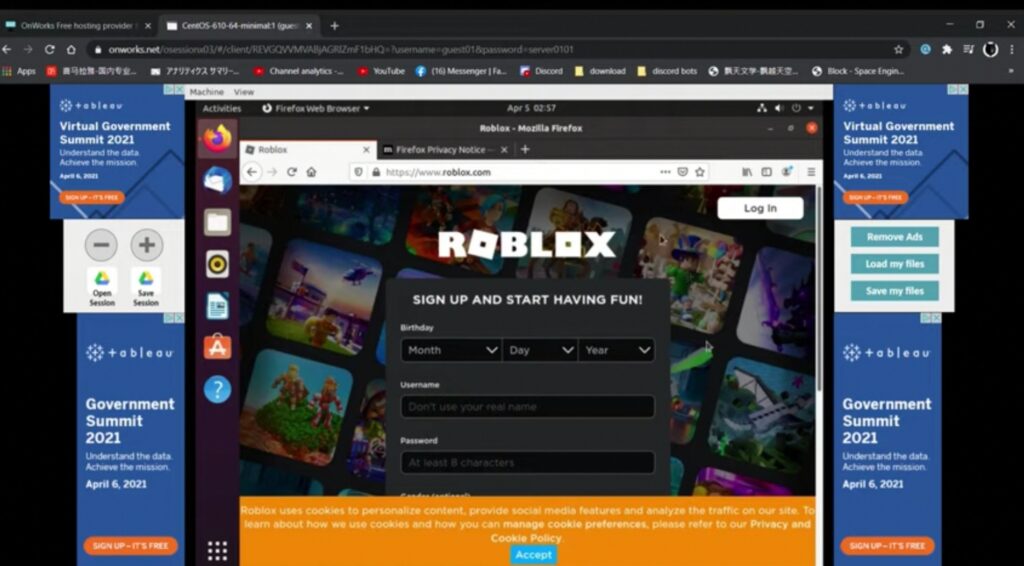A screenshot captures a desktop scene featuring a Chromium-based browser, likely Chrome, operating in dark mode. The browser window displays two open tabs at the top, each labeled in white font, though the specific tab titles are unreadable. Below the tabs, the address bar is visible, but its contents are too small to discern. Beneath the address bar resides a row of bookmarked websites, characterized by a mix of standard and Asian character titles.

Dominating the main part of the screenshot is a web page that appears to be a virtual machine interface overlaying the primary website displayed in the browser. Within the virtual machine window, there's an opened Firefox browser window showcasing the Roblox website, specifically targeting the sign-up page. The intricate layering indicates that the user is running a Firefox browser with the Roblox sign-up page within a virtual environment, all managed from their Chromium-based browser.